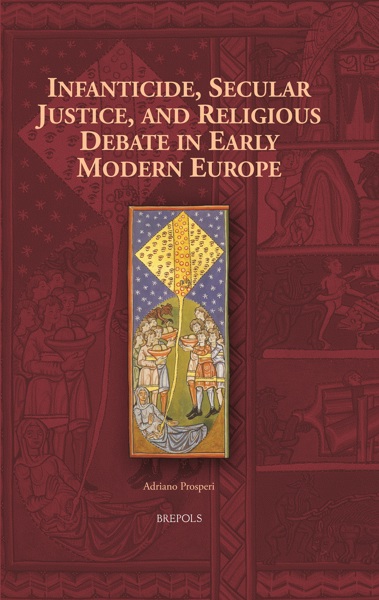The front cover of the book is adorned with a maroon or reddish-burgundy background featuring faint, ancient-looking illustrations of people in medieval European attire. These people appear to be engaged in various religious and social activities, holding baskets and wearing old-style clothing. Central to the cover is a vivid, tall rectangular illustration showing a scene where a person is lying on the ground, seemingly connected to a yellow kite, surrounded by onlookers holding bowls, possibly with fruits, suggesting some form of ceremonial act. The title, written above in a goldish or cream-colored font, reads: "Infanticide, Secular Justice, and Religious Debate in Early Modern Europe." The author's name, Adriano Prosperi, appears below the title, with the publisher listed as Brill.